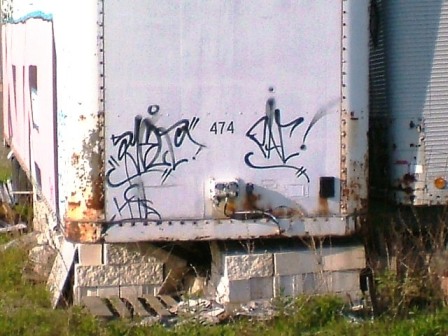This color photograph captures a bright, sunny day, showcasing a white trailer supported by light gray and broken cinder blocks, surrounded by light green grass. Beside the trailer stands a large light gray cylinder with ribbed sides, rivets, and an orange safety light, amidst patches of dead brown foliage. The trailer displays multiple instances of graffiti: a pink tag on the left side and black cursive writing on the backside against a white background. Near the center of the trailer, the number "474" is prominently visible. Despite noticeable rust on both sides, the image focuses on the black graffiti, which appears jumbled and evokes curiosity about its origins. Parts of another trailer peek from the right side of the frame, contributing to the overall urban and somewhat industrial scene.